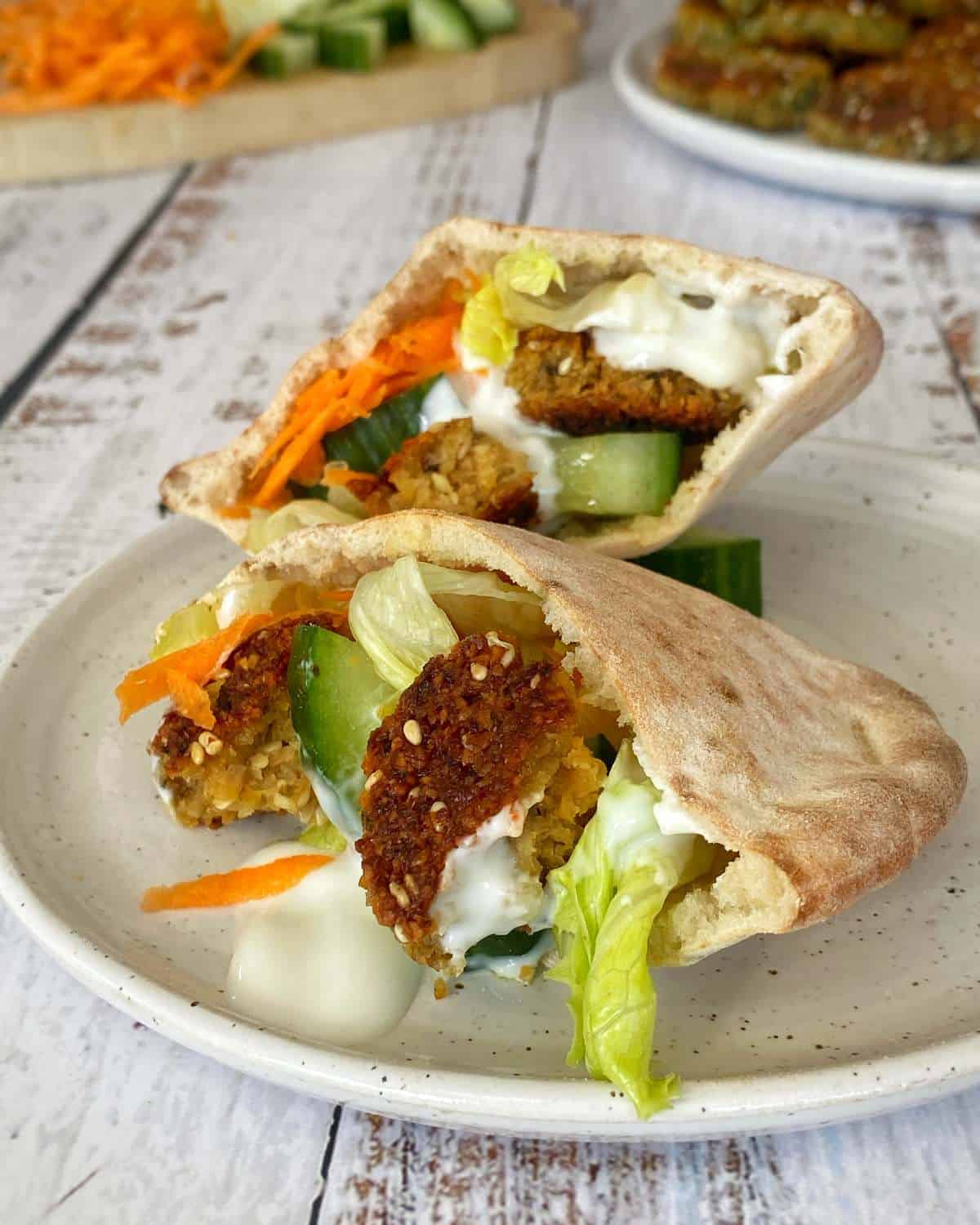This portrait-oriented image showcases a rustic, weathered white wooden table with patches of bare wood peeking through, creating a worn, antique look. Centered in the foreground is an off-white, black-speckled round plate featuring a pita sandwich cut in half. The pita, resembling a light brown tortilla, is loaded with vibrant ingredients: crispy falafel, shredded carrots, cucumber slices, lettuce, and a dollop of creamy white sauce, possibly ranch, with some drips visible on the plate. The sandwich halves are artfully positioned, one leaning against the other. In the upper corners of the image, additional food elements enhance the scene: the top left corner shows a light brown cutting board with carrot and cucumber slices, while the top right reveals another white plate heaped with more falafel pieces. The overall composition evokes a casual, country-style dining experience.